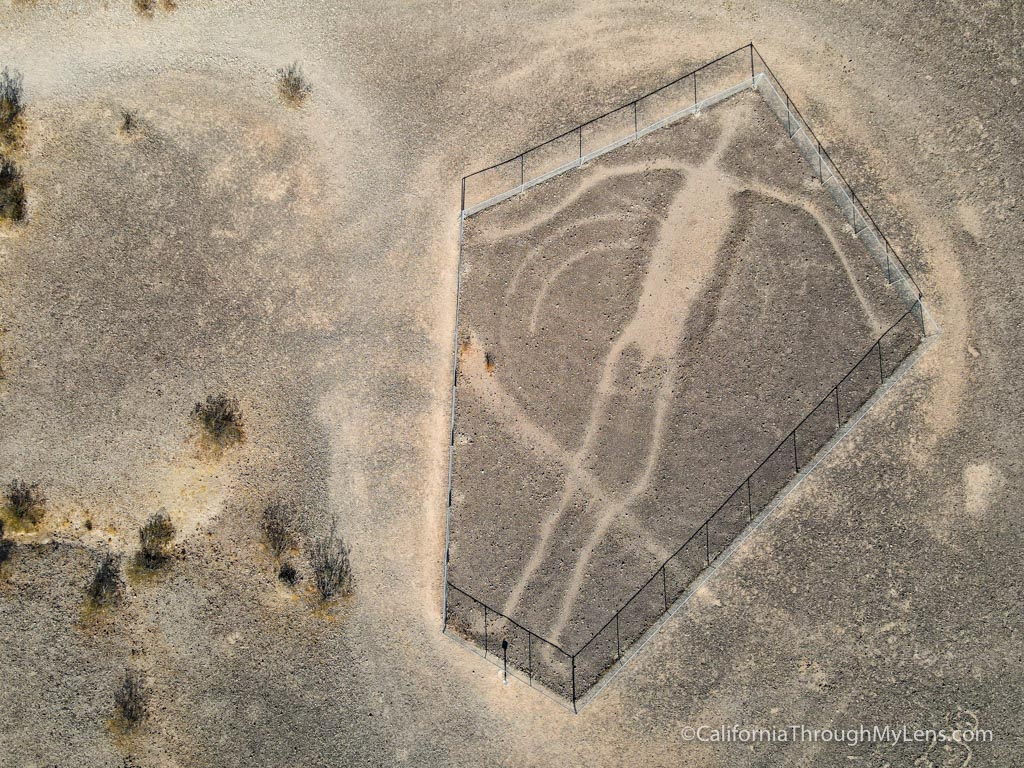This aerial view image, attributed to californiathroughmylens.com in the bottom right, showcases a pentagon-shaped fenced area in a mostly barren, dirt landscape interspersed with a few dried-out bushes. Inside the fence, a curious figure resembling an alien being is drawn. The figure features thin limbs, with one arm stretching towards the left and another towards the right, a small head at the upper right corner, and long legs extending downward. The fence, which starts at the bottom middle of the image, encloses this drawing with angled lines creating a pentagon whose sides vary in length. The ground inside and outside the fence appears dark brown, contrasting sharply with the lighter, tan lines of the alien figure. Surrounding the fenced area are tan and white swirls mixed with dark brown splotches, adding an otherworldly texture to the scene.